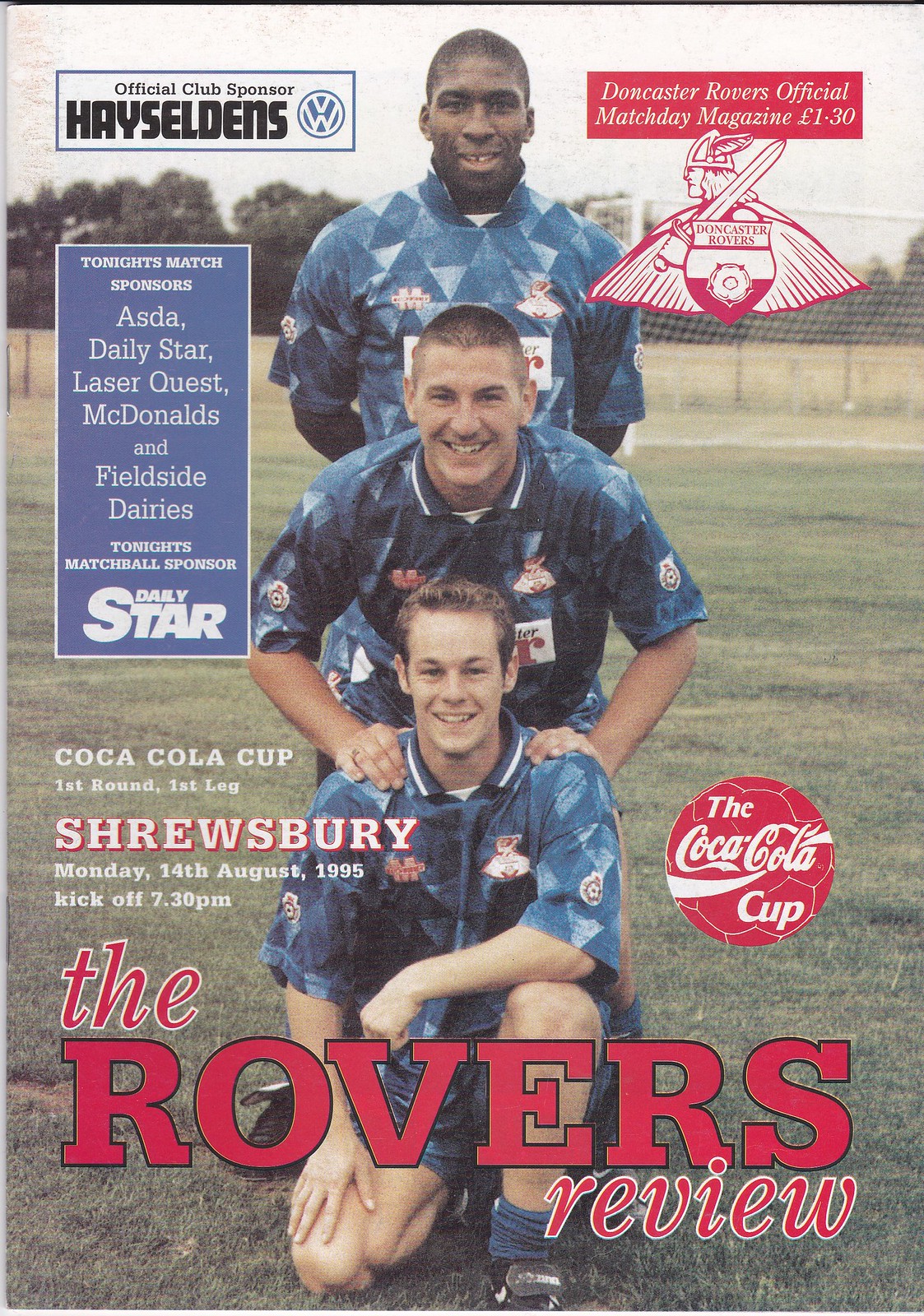The image is a detailed cover of the "Rovers Review" matchday program for a football (soccer) match. Central to the cover are three football players in blue uniforms. The front player, a Caucasian young man, is kneeling on one knee, smiling into the camera. Behind him, another Caucasian player is squatting with his hands on the shoulders of the kneeling player, also smiling. The third player, an African American, stands behind them with hands behind his back, smiling as well. The background features a football ground with goalposts, fences, and distant trees under a clear daytime sky.

In the upper left corner, the text reads "Official Club Sponsor, Hayseldens," next to the Volkswagen logo. The upper right corner features a red box stating "Doncaster Rovers Official Match Day Magazine, £1.30" below which is the Doncaster Rovers logo depicting a Viking warrior with a helmet, sword, cape, and shield.

A blue vertical rectangle on the left lists tonight's match sponsors: ASDA, Daily Star, Laser Quest, McDonald's, and Fieldside Diaries. It also names the match ball sponsor, Daily Star. Below, within this blue rectangle, the text details the event: "Coca-Cola Cup, First Round First Leg, Shrewsbury, Monday 14th August 1995, Kickoff 7:30 p.m."

Opposite on the right, there is a Coca-Cola Cup logo reinforcing the event's branding. At the bottom of the cover, the main headline reads "The Rovers Review" in large, red multi-shaped fonts.